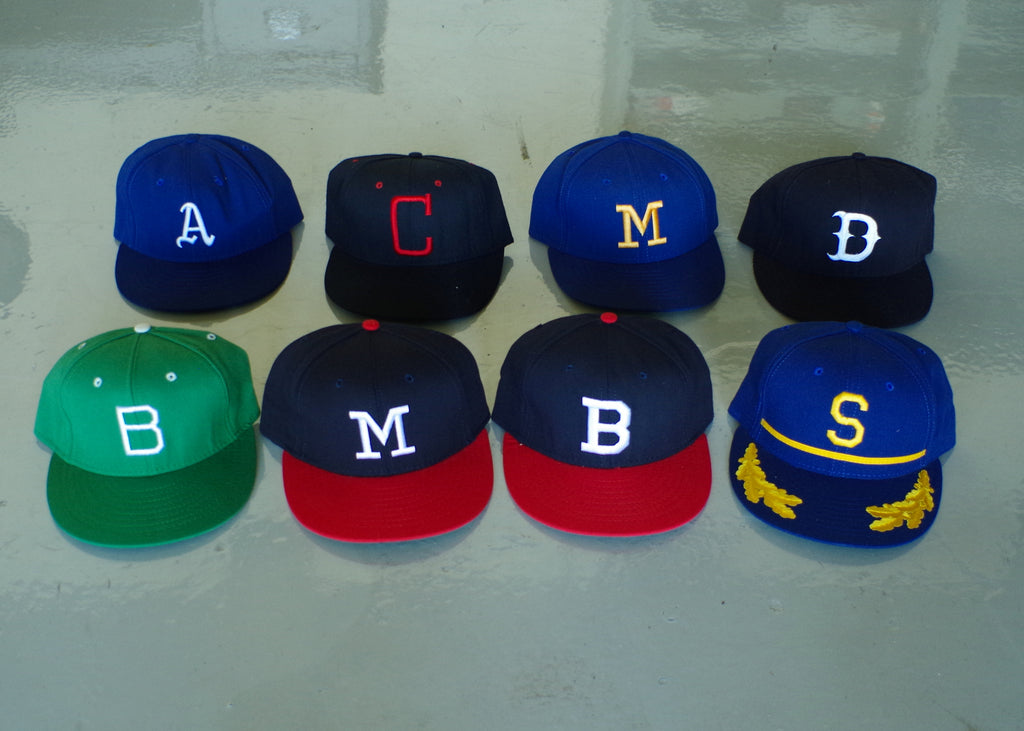The photograph showcases eight wide-brimmed baseball caps meticulously arranged in two rows of four on a reflective, light blue concrete floor. The surface subtly reflects furniture in the background, including a shelf and other indistinguishable items. Each cap is characterized by its own distinct color and monogram letter. 

From the top left, the first row features:
1. A blue cap with a white cursive 'A'.
2. A black cap with a red 'C'.
3. A blue cap with a yellow 'M'.
4. A black cap with a white 'D'.

In the bottom row, from left to right, the caps consist of:
1. A green cap with a white 'B'.
2. A blue cap with a red bill and a white 'M'.
3. A similar blue cap with a red bill, but featuring a white 'B'.
4. A blue cap with yellow laurels on the brim and a yellow 'S' underlined by a long line.